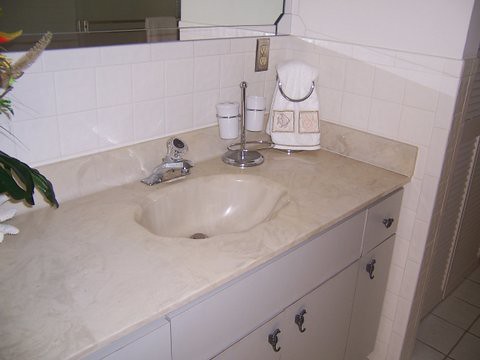The image showcases a meticulously organized corner of a bathroom. Central to the scene is a white cupboard with a sleek grey top adorned with metallic handles, exuding a modern aesthetic. Embedded in the worktop is a marble-look sink, complemented by a contemporary tap unit fixed against a modest splashback approximately six inches high. Above this, a taller, pristine white splashback extends upwards, enhancing the clean lines and minimalist design.

Within this well-arranged setup, a small towel rail stands on the countertop, cradling a neatly folded fabric hand towel. Adjacent to this, a silver-colored metal holder equipped with two containers—unidentified but potentially for toiletries or other bathroom essentials—features a circular design on its front face. Adding a touch of intrigue, a small brown plaque is affixed to the splashback, though its purpose remains unclear.

A mirror, securely mounted above the basin, reflects the simple elegance of the space, while a plant with long, fuzzy, and soft-looking flower or seed heads peeks into the frame from the left-hand side, introducing a hint of nature. The overall ambiance of the bathroom corner is one of spotless cleanliness and refined simplicity.